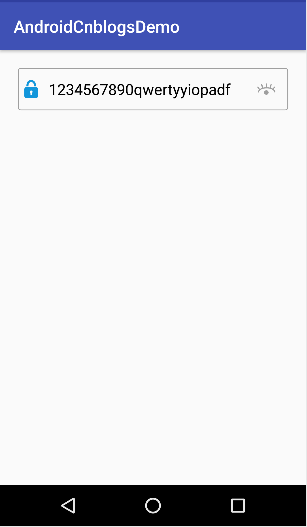This screenshot appears to be taken from an Android phone, as indicated by the navigation icons at the bottom of the screen: a left-pointing arrow for the "Back" function, a circle for the "Home" function, and a square for accessing recent apps. The overall appearance is quite generic and predominantly gray, signifying a lack of customization.

At the top of the screenshot, there's a blue strip containing white text that reads "ANDROIDCNBLOGSDEMO." Below this header, there is a white rectangular input field, likely intended for entering a password. This field is accompanied by a blue lock icon on the left, indicating that it is active or currently selected. On the right side of the input field, there's an eye icon, which suggests that tapping it would toggle the visibility of the entered text, allowing the user to see the password instead of asterisks.

In this particular screenshot, the input field contains a series of numbers and letters: "1234567890QWERTYOILPADF," which seems to be a placeholder or demonstration text illustrating how the app works rather than an actual password.